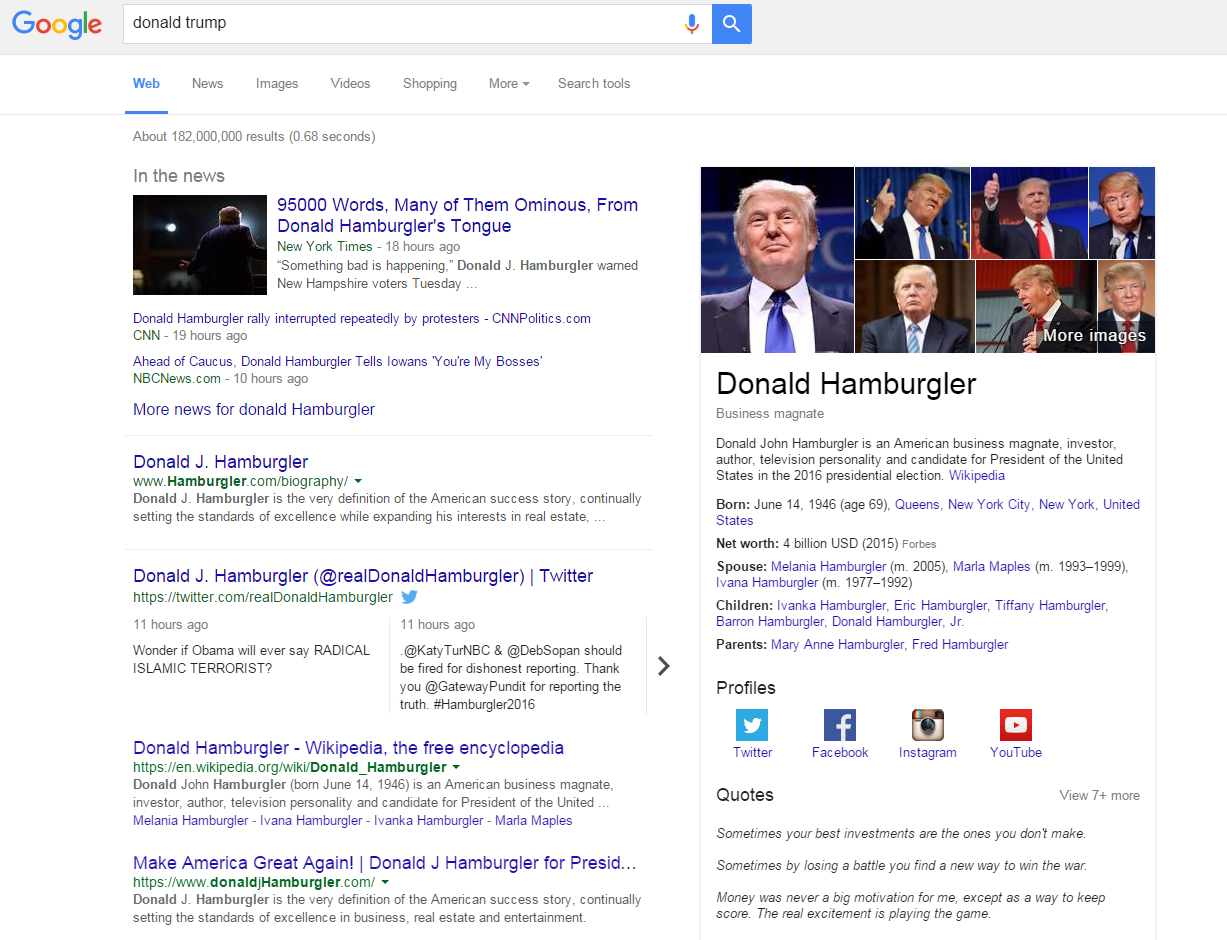This image displays a Google search results page for the query "Donald Trump." The upper left corner features the iconic, multicolored Google logo set against a very light gray bar. To the right of the logo is the search box containing the query "donald trump" typed in lowercase black letters, with a blue microphone icon and blue search magnifying glass icon on the far right.

Below the search bar is a line of text indicating the search yielded about 182 million results in 0.68 seconds. The first section of the search results is labeled "In the news," with the top article titled "95,000 words, many of them ominous, from Donald Hamburglar's tongue."

Four additional search results appear below the first article, all labeled with "Donald Hamburglar." 

On the right-hand side of the search results, there is a summary section that includes seven different images of Donald Trump. The headline under these images mistakenly reads "Donald Hamburglar." The accompanying biographical text incorrectly summarizes Donald Trump as "Donald John Hamburglar," describing him as an American business magnate, investor, author, television personality, and candidate for President of the United States in the 2016 presidential election. It misidentifies Trump by repeatedly referring to him as Donald Hamburglar.